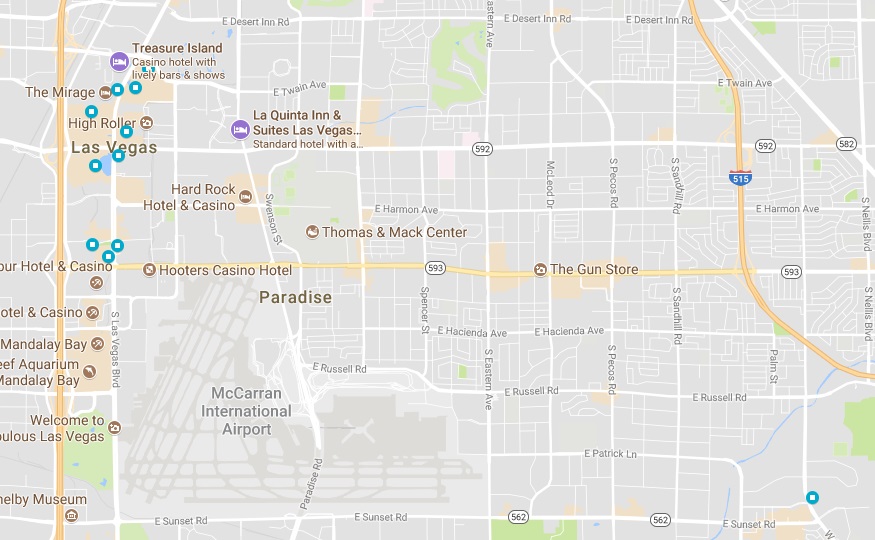This is a detailed screenshot from a mapping application, likely Google Maps or Apple Maps. The map is crisscrossed with a network of white roads, ranging from main thoroughfares to narrower alleyways, driveways, and parking areas. A prominent, thicker road, shaded in a darker, peachish-orange hue, runs vertically from the top to the bottom of the image, entering about an inch from the left edge.

Just to the right of this main road, clusters of blue circles containing light blue squares can be seen, which likely indicate hotels. Another slightly thinner road intersects this primary route horizontally in the middle section of the map. This road takes a slight downward angle to the right approximately two inches from the right edge before exiting the frame. It also continues upward, angling slightly left around two inches from the top before it too leaves the visible area.

Below the horizontal road, aligned to the right of the vertically running main road, there are four brown circles with some kind of emblem inside; these represent casinos. Near the top, just to the right of the main vertical road, are two notable landmarks. About an inch down from the top is a purple marker labeled "Treasure Island," and diagonally down to the right, another purple marker signifies "La Quinta Inn & Suites Las Vegas."

Toward the bottom section of the map, near the cluster of hotels, there's a significant area labeled "McCarran International Airport." This label appears as you move right from the hotels and then slightly downward, indicating the airport's location relative to other features on the map.